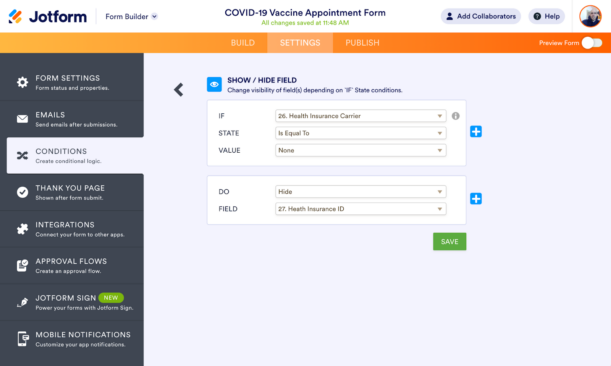The screenshot captures a detailed view of the JotForm Form Builder interface, oriented in landscape, making it suitable for tablets, laptops, or desktop computers.

At the top of the screen, the JotForm logo is prominently displayed in blue, red, yellow, and black colors, with an accompanying down arrow and the text "Form Builder." Below the logo, the header indicates that a "COVID-19 Vaccine Appointment Form" is being edited, with a green note confirming all changes were saved at 11:48 a.m.

On the top-right corner of the interface, there are two icons. The first is a gray bubble with a person symbol, labeled "Add Collaborators." Adjacent to it is another gray bubble featuring a black circle with a question mark, labeled "Help." Further to the right, a circular icon displays a woman's face.

Directly beneath this upper section, an orange navigation bar houses three tabs: "Build," "Settings," and "Publish," with the "Settings" tab currently selected. To the far right of this bar, viewers can see the "Preview Form" option accompanied by a toggle switch, which is currently turned off.

On the far left side of the interface, a black column includes various settings options, each represented by an icon and text:
- A gear wheel for "Form Settings," encompassing "Form Status" and "Properties."
- An envelope labeled "Emails."
- An item with text that is partially unreadable due to small font size.
- A gray bar indicating the currently selected "Conditions" option, represented by an "X" shape.
- A white circle with a check mark, labeled "Thank You Page."
- A puzzle piece for "Integrations."
- A page icon with a circle and check mark for "Approval Flows."
- A quill pen next to "JotForm Sign," noted as "New" with a green oval.
- An image of a smartphone with an overlay symbol for "Mobile Notifications."

The main section of the website displays several functional elements for condition settings. It begins with a left-facing arrow and a blue box featuring an eye icon and the words "Show/Hide Field," explaining the function to change field visibility based on state conditions.

Below this, there are two white boxes:
1. The first box is labeled "If," with a dropdown menu set to "26, Health Insurance Carrier," which can be modified. The condition "State is equal to value none" is specified, with a blue plus-sign button on the far right.
2. The second box is labeled "Do," where "Hide" is selected. It specifies the field "27 Health Insurance ID," with another blue plus-sign button on the far right.

Below these boxes, there is a prominent green button labeled "Save."

Overall, the screenshot provides a comprehensive view of the various tools and settings available within the JotForm Form Builder.